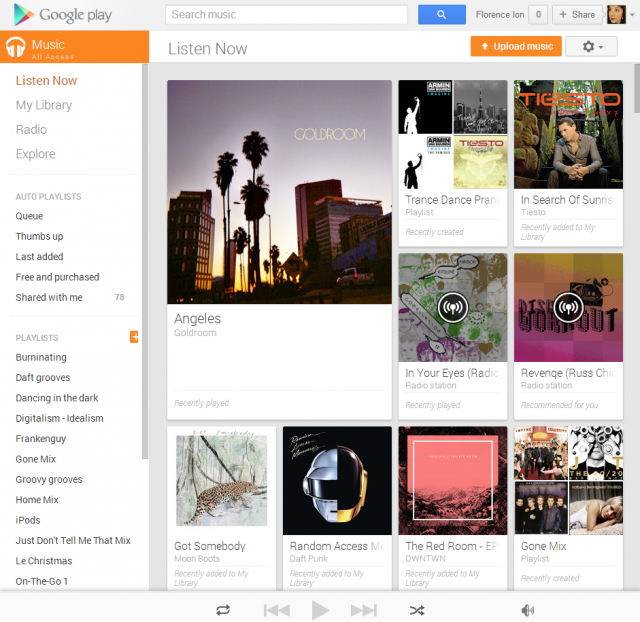The Google Play landing page is set against a light gray background, providing a clean and minimalist interface. In the upper left-hand corner, the recognizable Google Play icon is situated alongside the words "Google Play" in gray text. Directly to the right is a search bar with the placeholder text "Search Music." Adjacent to the search bar is the user's profile picture.

Below the Google Play heading, a vertical navigation menu is prominently displayed. The first option, "Music," is highlighted in orange, indicating it's the currently selected section. The submenu item "Listen Now" is also highlighted in orange, denoting its active state. Below this, the menu lists options in gray text: "My Library," "Radio," "Explore," "Auto Playlist," "Cue," "Thumbs Up," "Last Added," "Free and Purchased," and "Shared with Me." Following these are user-specific playlists, including titles such as "Berninating," "Daft Grooves," "Dancing in the Dark," "Digitalism Dash Idealism," "Franken Guy," "Gone Mix," "Groovy Grooves," "Home Mix," "iPods," "Just Don't Tell Me That Mix," "Le Christmas," and "On the Go 1."

To the right, at the top of the main content area, the "Listen Now" section is heading the page, featuring several video thumbnails. These thumbnails include a range of playlists and recently accessed items: "Angelus Gold Room," "Trance Dance Party Playlist," "Recently Created," "In Search of Sunrise," "Recently Added to My Library," "In Your Eyes," "Recently Played," "Revenge Recommended for You," and several other curated selections. Each thumbnail is visually distinct, offering the user immediate access to their personalized music content.